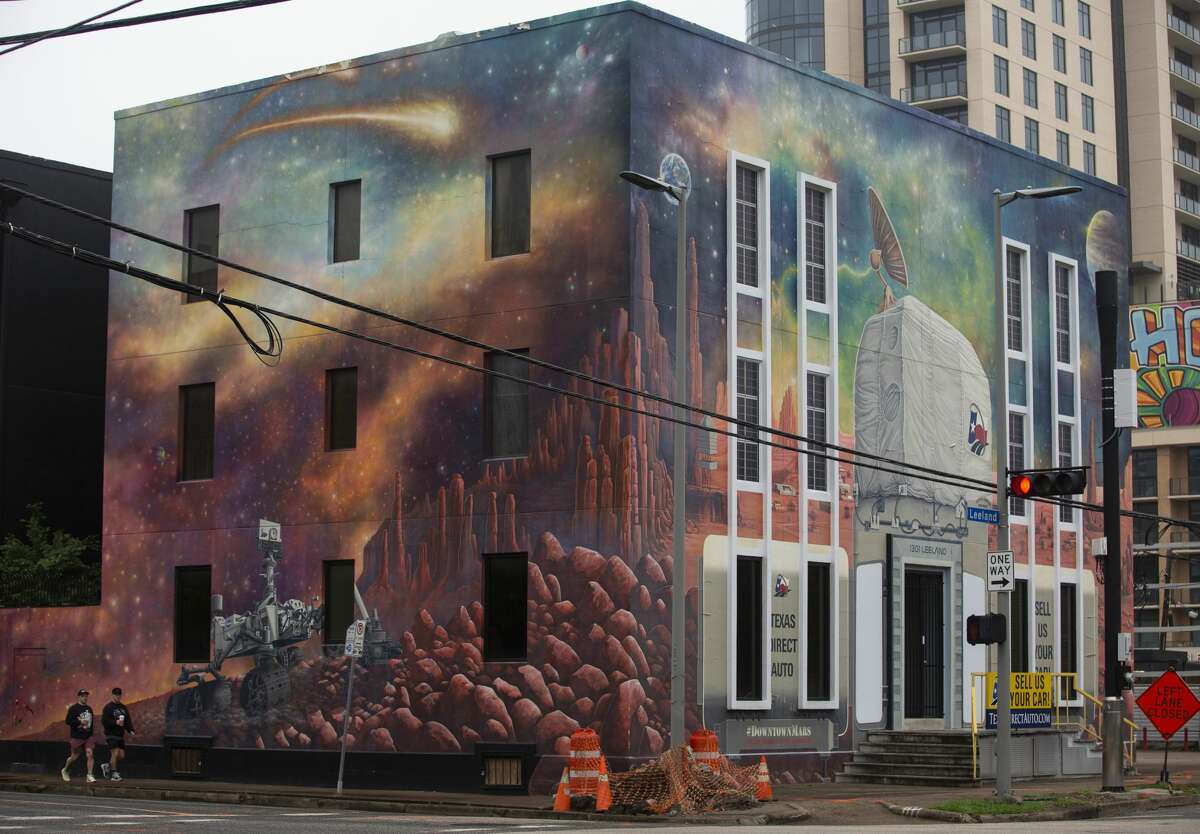This photo captures a vibrant street corner in a bustling metropolitan city. The focal point is a three-story building, adorned with a striking, colorful mural that transforms its flat walls into an otherworldly scene. The mural depicts a nebula on an unexplored planetary landscape, featuring celestial elements like shooting asteroids, planets, and distant stars as well as an array of space instruments and robots, reminiscent of a NASA habitat on an asteroid. The entrance of the building, enhancing the mural's effect, is cleverly integrated into this cosmic scene. Above the entrance, signs read "Texas Direct Auto" and "Sell Us Your Car," indicating it’s an auto-related business.

In the foreground, city elements populate the scene, including a one-way street sign, construction signs, cones, netting, and various cables running along the sidewalk. Two pedestrians, dressed in casual attire—shorts, tennis shoes, and black tops—are seen walking past the building. Their attire suggests either two men or possibly a man and a woman, both in relaxed, athletic clothing. The overcast sky casts a diffused light over the scene, further highlighting the mural's vivid colors.

In the background, there stands a significantly taller, plain tan building that appears to be either a hotel or an apartment complex, characterized by its numerous balconies. This towering structure contrasts sharply with the artistic three-story building in the foreground. The street corner is also marked by construction activity, including an orange sign stating "Left Lane Closed" and barriers to guide pedestrians safely around the site, lending a sense of urban dynamism to the overall scene.